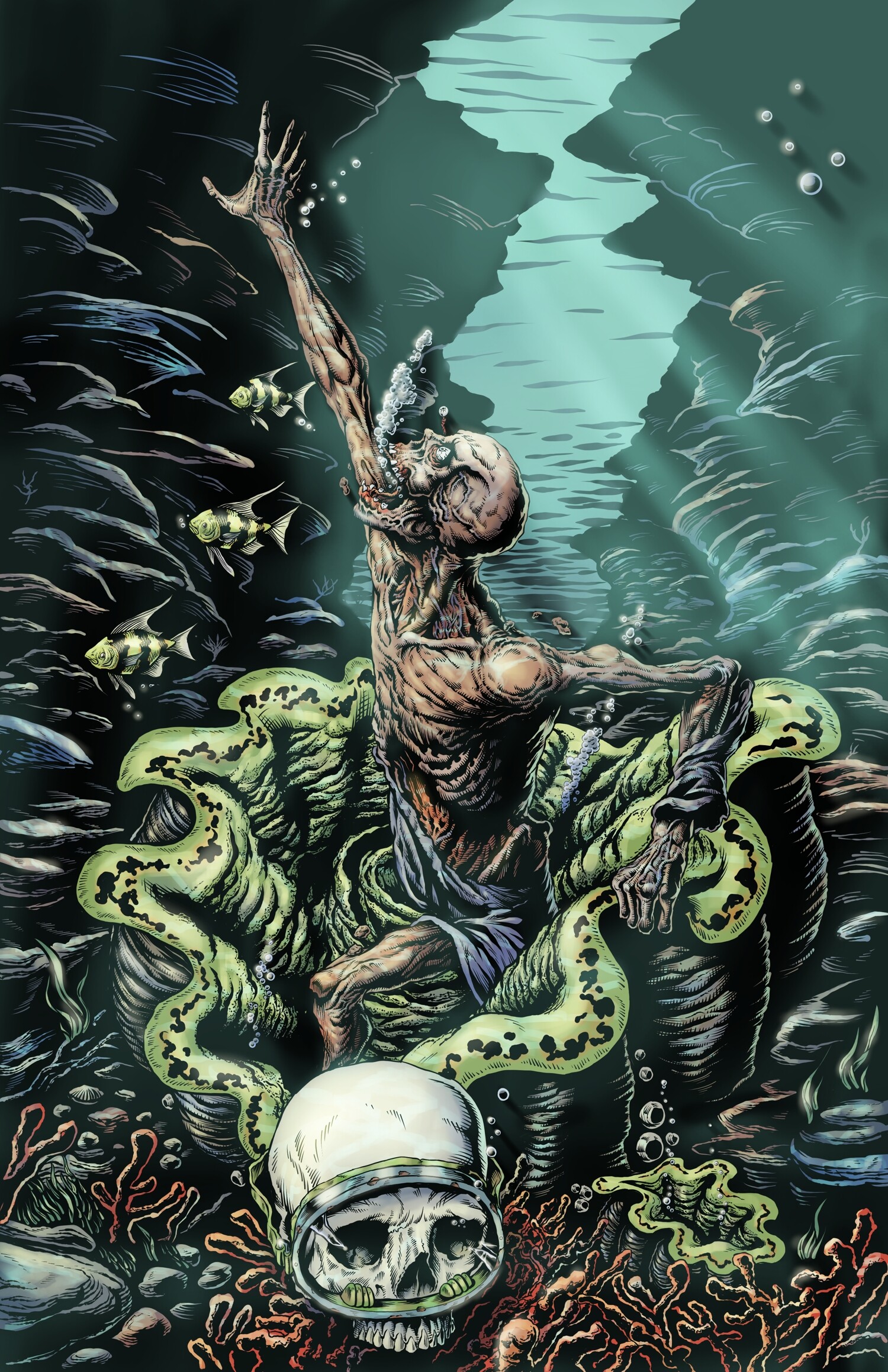This captivating and somewhat eerie artwork depicts a decaying human figure emerging from a chaotic underwater scene, characterized by a contrasting palette of black, gray, sea green, blue-green, lime green, and white. The central figure, a skeletal creature with remnants of muscle, is posed dramatically with its right arm outstretched towards the surface, its mouth open as if in a scream of desperation. The man’s head is turned to the left, capturing a moment of terror and urgency. At the base of the scene lies another striking detail—a whitewashed human skull donned in scuba goggles, partially buried in the rubble and debris that clutter the seabed. Surrounding this skull are elements of underwater life, including dark coral and sea urchins. Adding to the otherworldly atmosphere are lime green, octopus-like arms that encroach from behind. The background features a narrow, light bluish-green waterway, bordered by banks colored in hues of green, black, and white, suggesting a confined aquatic environment. The overall composition is further enhanced by light streaming down from the water's surface, penetrating through stone caves, and casting an eerie glow over the haunting scene below.